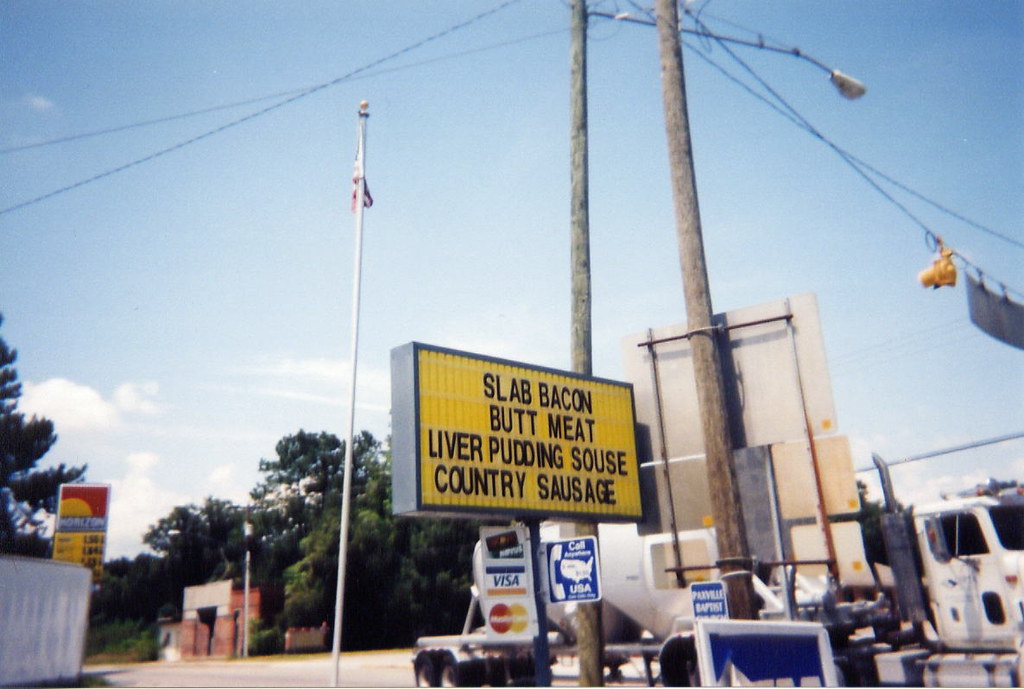This vibrant daytime photograph captures a gas station scene bathed in clear blue skies adorned with white, puffy clouds, primarily visible towards the top left. A central feature of the image is a yellow sign with a black frame and text promoting slab bacon, butt meat, liver pudding, sous, and country sausage, accented by Visa, MasterCard, and Discover logos beneath it. Adjacent to this sign, a blue "Call USA" sign is also evident, accompanied by a small image of a phone icon. A white flagpole with an American flag stands to the left, while to the right, a tall wooden pole equipped with a light and festooned with power lines extends upward.

In the background, to the left, trees partially obscured by the overhanging clouds line up behind a red and yellow gas station sign, its gas prices too blurry to decipher. A reddish-bricked building that appears old and unoccupied sits towards the back right of the image, with its light gray concrete top visible. Below these structures lie additional details: a white wall in the bottom left corner, the yellow traffic light housing at the top right, and a conspicuous white concrete truck in the bottom right. Scattered throughout the scene are numerous black cables and power lines, intertwining above the diverse elements of this roadside tableau.